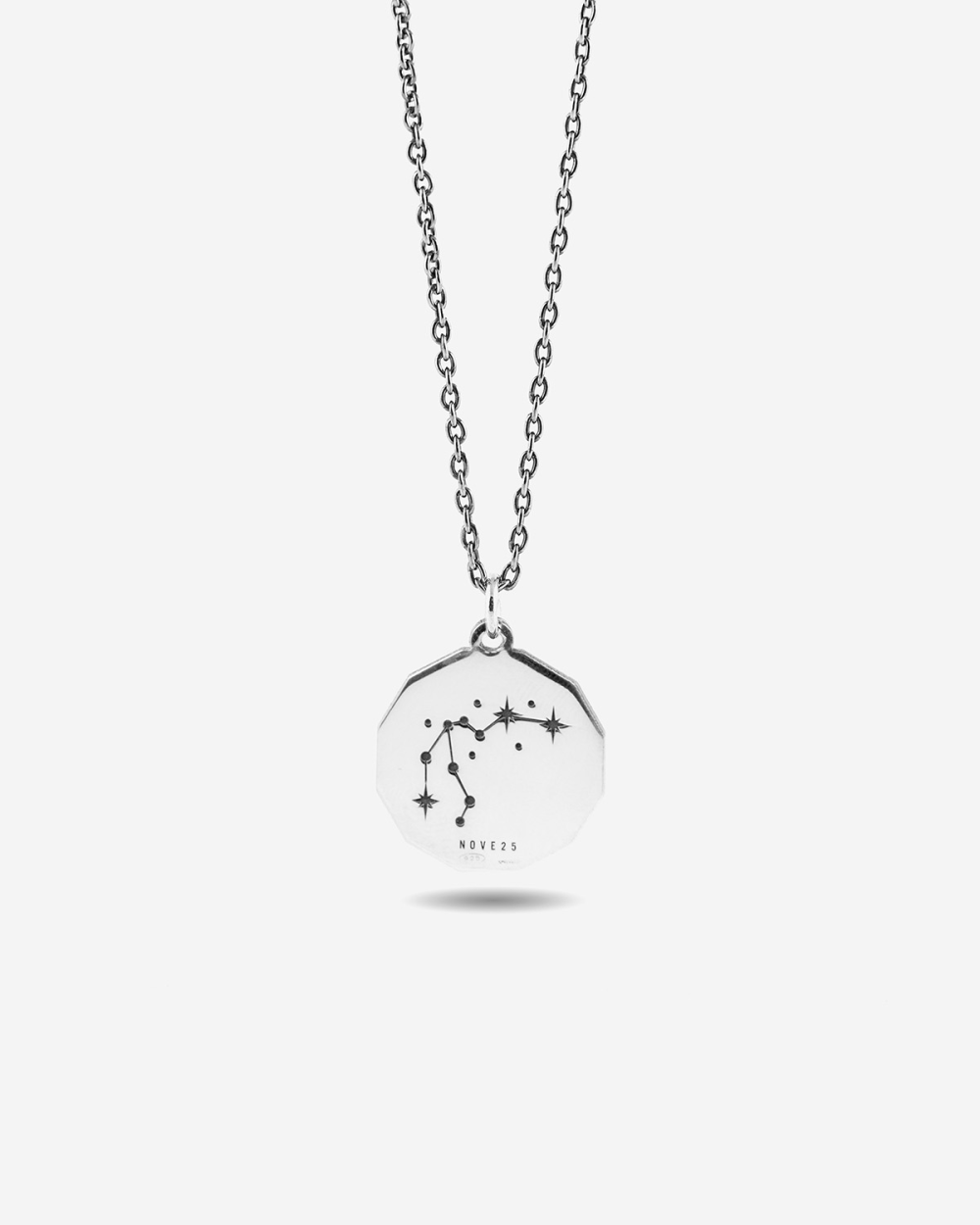The image features a silver necklace against a simple, off-white to light gray background. The necklace has a delicate, small link chain that is likely made of sterling silver, platinum, white gold, or stainless steel. The focal point of the necklace is its octagon or hexagon-shaped pendant, which is engraved with a constellation-like design. The constellation is depicted using lines connecting various points, with some points highlighted to indicate star bursts. Below the celestial pattern, the inscription "NOVE25" is visible, possibly denoting the name of the constellation or the brand of the necklace. The image is monochromatic, emphasizing the pendant, which appears to be floating and not touching the ground, with no other distracting elements in the foreground or background. The pendant is about the size of a quarter, suitable for any gender to wear.